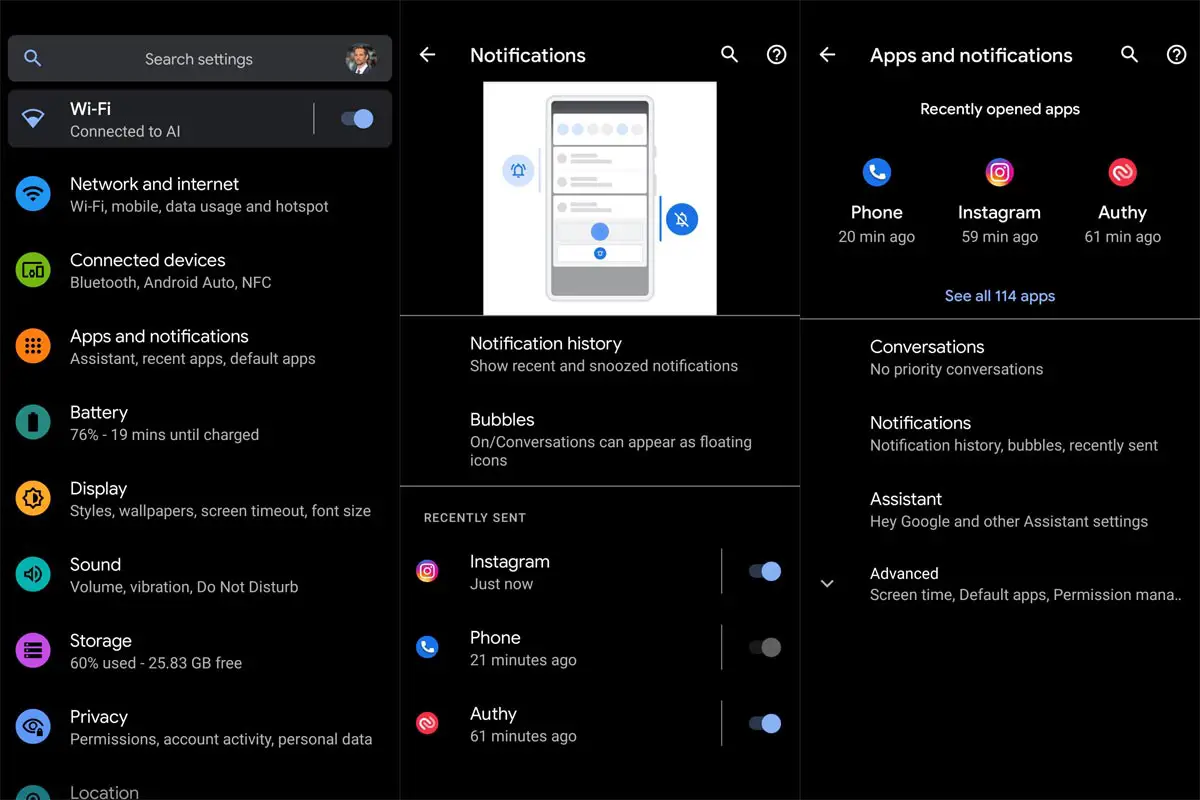This screenshot showcases a computer screen displaying a settings menu, predominantly set against a black background. Various sections are delineated by colorful icons, adding vivid contrast to the otherwise dark interface. 

On the left side of the screen, there are several icons each representing different settings categories. These include:
- A blue circle with a white phone icon for the "Phone" settings.
- The vibrant blend of yellow, pink, and bright colors symbolizing "Instagram." 
- A red circle with two interlocked C's for what seems to be "Arthy" or "Athy."

On the right side, you can spot a couple more icons:
- The traditional Wi-Fi symbol coupled with the label "Wi-Fi."
- A blue circle mirroring the shape of Wi-Fi for the "Network & Internet" section.

At the top of the screen, there is a profile picture followed by a search bar labeled "Search Engine." Below, a vertical list of additional settings categories is visible:

- Wi-Fi
- Network & Internet
- Connected devices
- Apps & notifications
- Battery
- Display
- Sound
- Storage
- Privacy
- Instagram
- Phone
- Arthy/Athy

The arrangement provides a comprehensive yet visually structured view of various device settings.